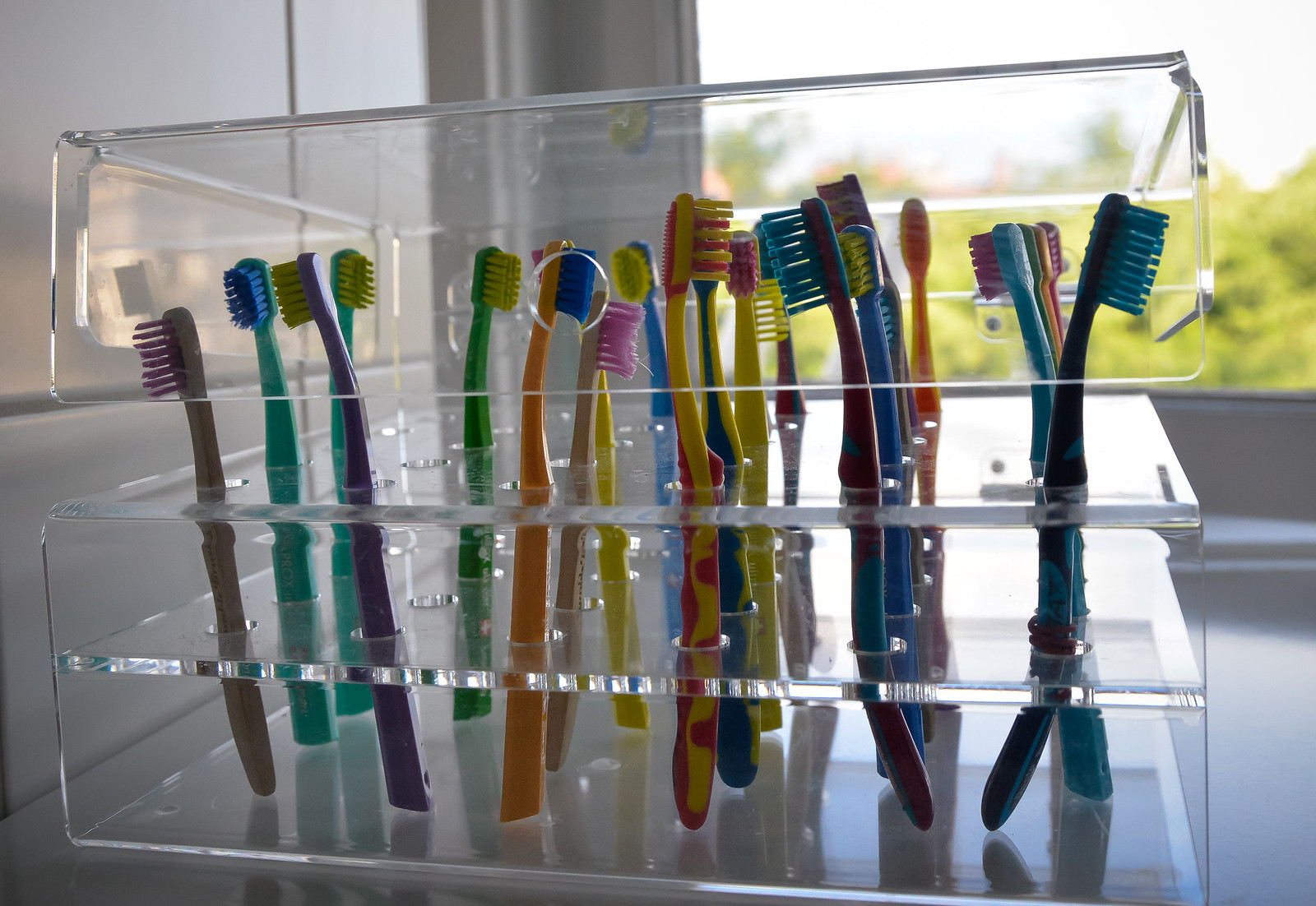This image captures a side view of a collection of colorful, manual toothbrushes of various sizes and designs, all housed in a large, transparent plastic toothbrush holder. The holder, resembling a clear plastic box, is set on a glass surface and features a multi-layered design with two levels, each pierced with circular holes to hold the toothbrushes upright. The toothbrushes, which range in color from red and yellow to orange, green, and blue, are inserted haphazardly in different orientations, some facing the right, left, or towards the camera. The holder is topped with a clear, somewhat floating lid, and its sides are partially open to the air. The room in which the toothbrush holder sits is minimalistic with white walls and a spacious design. In the background, an out-of-focus window reveals a daytime view of blurry trees, contributing to a serene and uncluttered atmosphere.